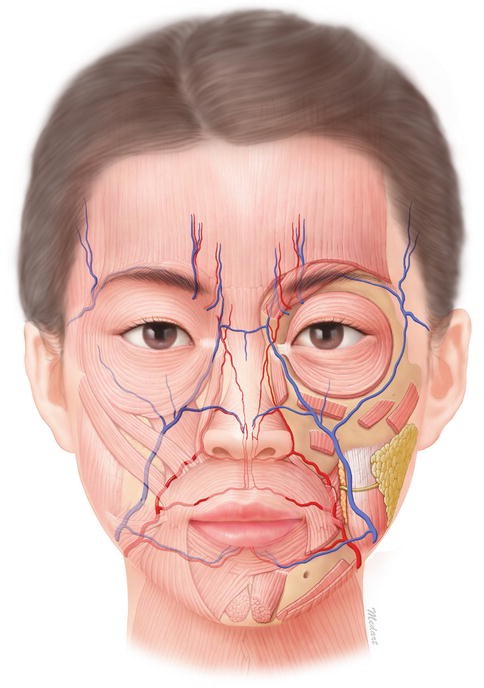This image is a detailed anatomical diagram of a human face. The individual has brownish hair pulled back from their face, making it ambiguous whether they are male or female. They have dark eyebrows and reflective brown eyes, framed by small ears. The skin tone is a light shade of tan, and the expression is very serious, with no hint of a smile.

The diagram vividly illustrates various layers beneath the skin. Prominent blue lines, likely representing veins, circle one eye, extend up the nose, and spread across the face. In addition, red lines and pink patches depict tendons or muscles, adding to the complexity of the facial structure. Some areas, such as the ears and sides of the face, display regular skin, while other sections reveal underlying layers, including a brown layer that might represent deeper tissue or muscle.

This stark representation of facial anatomy, showing veins, sinuses, tendons, and muscle directions, provides an insightful look at how these elements interlace beneath the surface. The overall effect, although somewhat unsettling, offers a fascinating glimpse into the intricate workings of the human face.